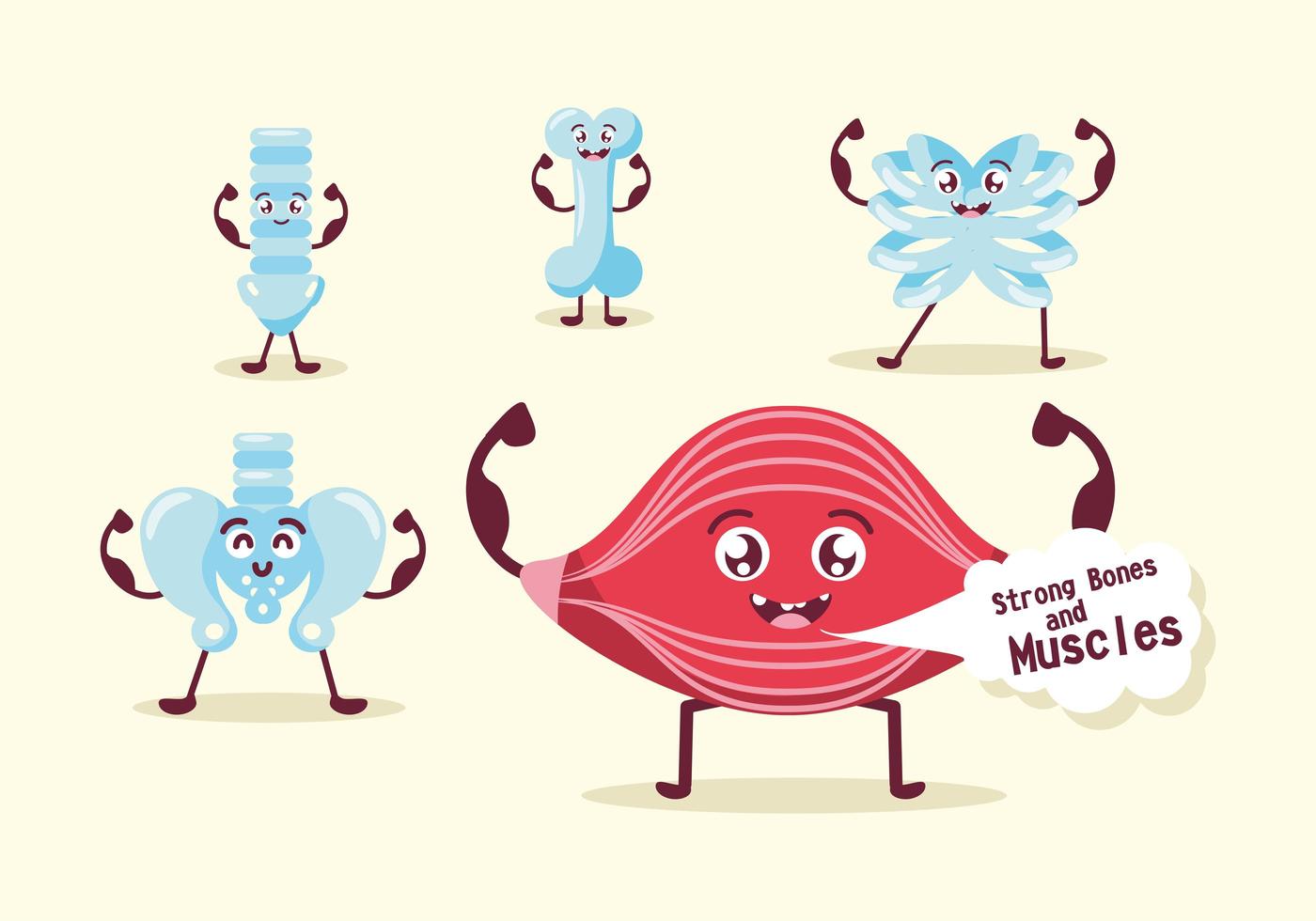This vibrant and cheerful poster promotes strong bones and muscles, making it perfect for an elementary audience. Featuring cartoon-style artwork, the poster displays five distinct bones in blue, each with expressive faces, arms raised as if flexing muscles, and sporting wide smiles. The bones depicted include a hip bone with kidney-shaped formations, various vertebrae resembling a lower spine, a circular ribcage with ribs extending outward, and a milk bone-shaped femur.

Amidst these blue characters, the illustration also showcases a prominent red figure representing a muscle (frequently mistaken for a red blood cell or a red M&M by kids due to its design). This character, larger than the others, is an oval shape adorned with vein-like markings in shades of red and pink. It too has a friendly smile, big eyes, arms, and legs.

The backdrop of the poster is a light yellow, enhancing the playful and engaging feel of the graphic. Concluding the message is a speech bubble emerging from the red figure's mouth, stating in bold, dark brown text on a white background: "Strong Bones and Muscles." This delightful illustration effectively communicates its health message in a fun and memorable way.